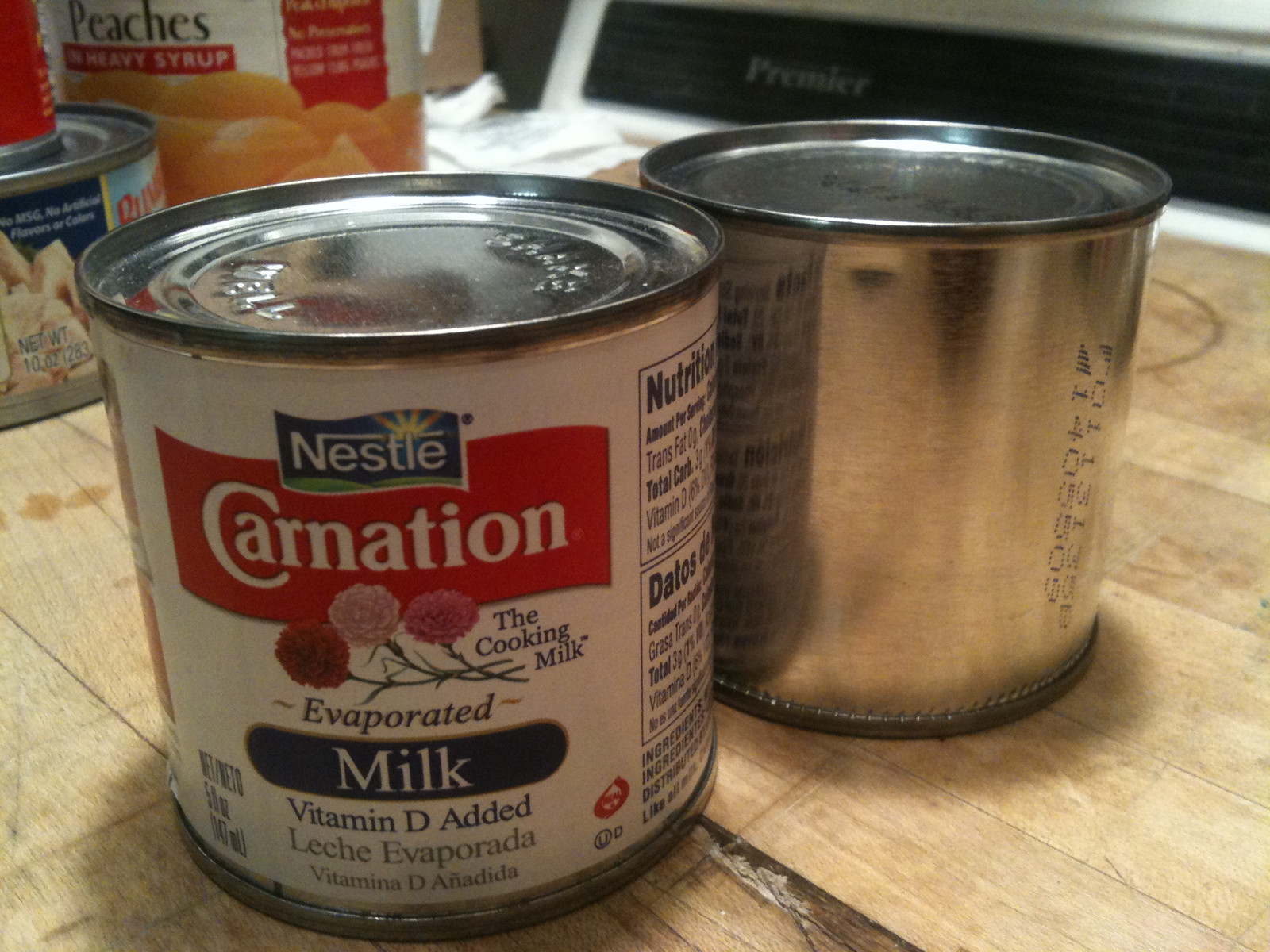The photograph, taken indoors likely in a kitchen, showcases a light-colored wooden table as the primary setting. The focal point of the image is a collection of cans arranged on the table. Dominating the foreground, a silver, unlabeled can marked only with black serial numbers stands out starkly. Positioned nearer to the camera and adjacent to the silver can is a Nestle Carnation evaporated milk can, distinguished by its predominantly white label accented with red and blue hues. The label prominently reads "The Cooking Milk" and "Vitamin D Added" along with bilingual text "Leche Evaporada" and "Vitamina D Añadida." Part of the nutrition facts is also visible on the side of this can. In the background, additional cans can be seen, including a can of peaches. However, the label of another can next to the Carnation milk is obscured, making it undiscernible. The composition and arrangement of the cans draw attention to the details of their labels and packaging, emphasizing the Nestle Carnation evaporated milk can as a key element in the scene.